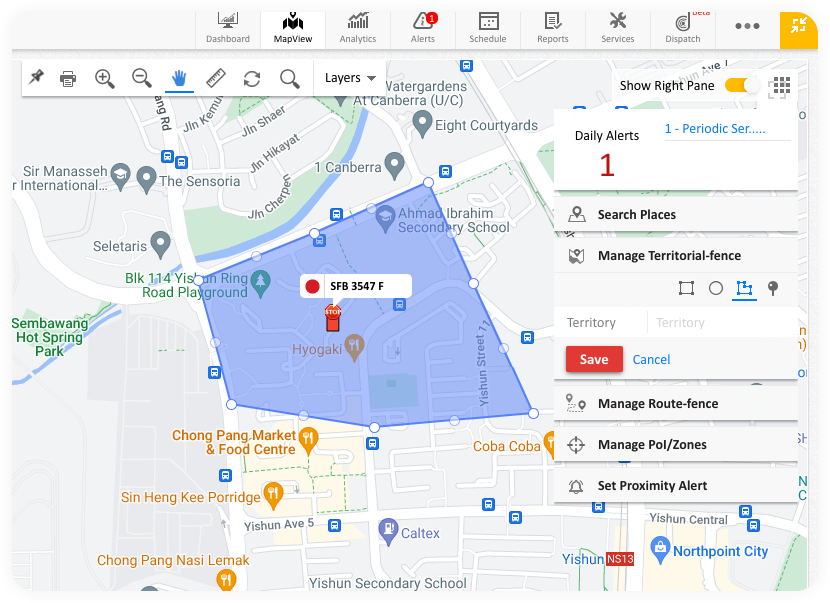The image depicts a comprehensive interface of a square map with multiple functional layers and icons. At the top, there is a horizontal toolbar featuring various navigation and management options labeled from left to right: Dashboard, Space Map View, Space Analytics, Space Alerts, Space Schedules, Space Reports, Space Services, Space Dispatch. Following these labels, there appear to be three ellipsis dots and a square icon with rounded corners on the right, possibly for screen maximization.

Below this toolbar rests a secondary navigation strip, laid out on a rectangular bar, encompassing a push pin icon for pinning, a printer icon for printing, and a magnifying glass icon for zooming in or out of the map. Notably, this strip includes an underline under a blue hand icon, distinguishing it from the other green-colored icons. 

Moving to the main area of the interface, there is a small square icon displaying a bus silhouette inside either a black or blue square, labeled "Show Right Pane." Beneath this, under a section titled Daily Alerts, the numbers "1" and "1 - Periodics" are listed with ellipsis following them, indicating the presence of additional data or options.

The focal point of the map highlights a specific location, marked by a red vertical rectangle with a prominent round stop sign reading "STOP." Above this stop sign, a speech bubble denotes "SFB3547F," which is presumably the destination code the map is concentrating on.